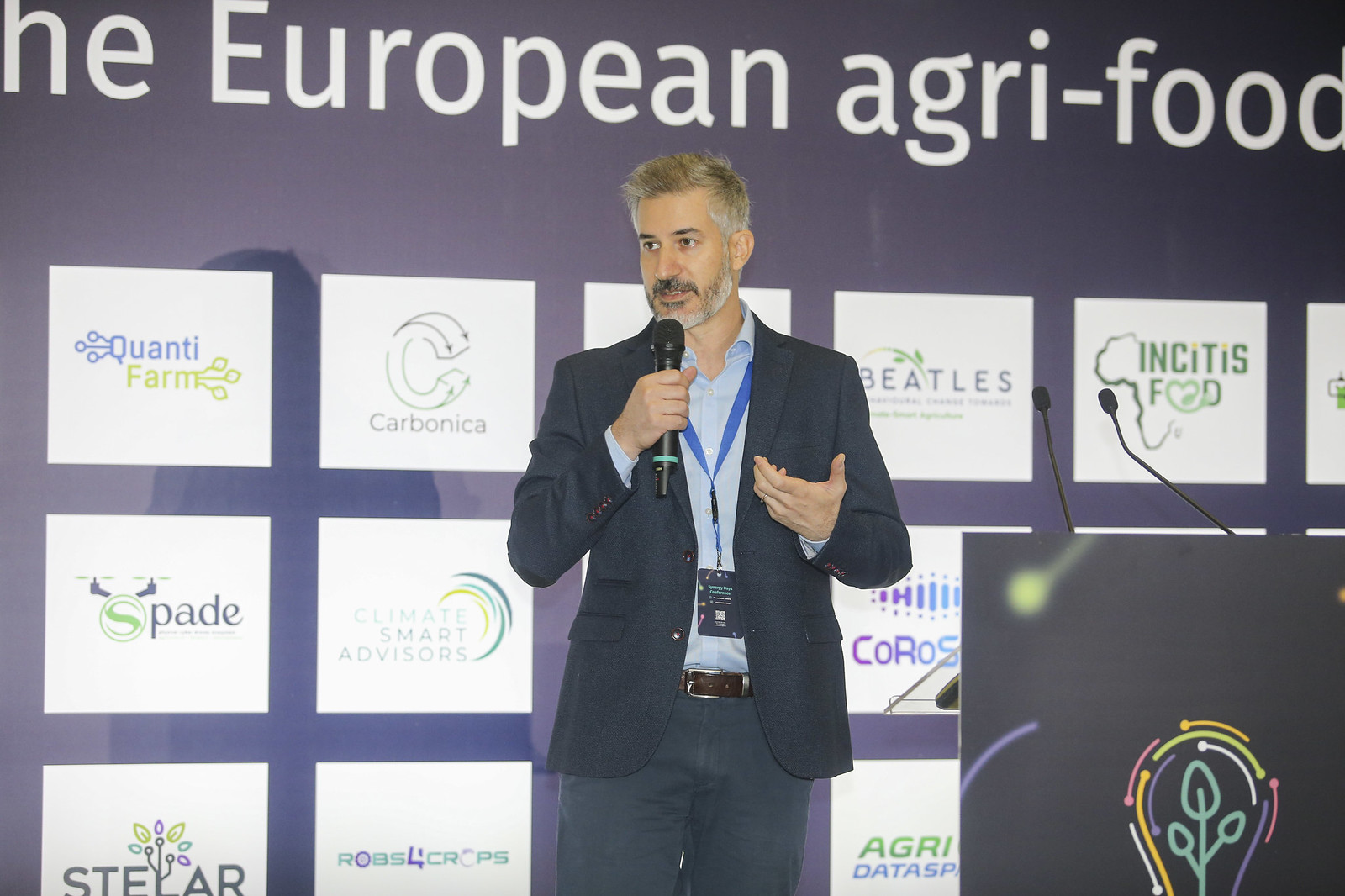In the color photograph, a middle-aged man is captured mid-speech at a conference, likely an agricultural or climate convention. He stands on stage with a blue wall behind him, featuring the partially visible text "the European agri-food" at the top. Below this text, there's a grid of white squares displaying various organization logos, such as Quantifarm, Carbonica, Spade, Stellar, Insitus Food, Robo for Crops, Climate Smart Advisors, and more, some of which are obscured by his presence.

The man, who appears to be in his 40s or 50s, has short, graying hair, a dark mustache, and a light-colored beard. He is dressed in a dark blue suit jacket over a light blue button-down shirt, with matching slacks and a brown belt. A blue lanyard with a name tag or ID hangs around his neck. He is holding a black microphone with a green band near its base in his right hand, which he has raised to his mouth as he speaks, emphasizing his engagement with the audience. 

To his right, just off-center in the image, stands a podium adorned with a black card that features an artistic depiction of a light bulb with a plant growing inside it, symbolizing innovation and growth, flanked by two microphones.